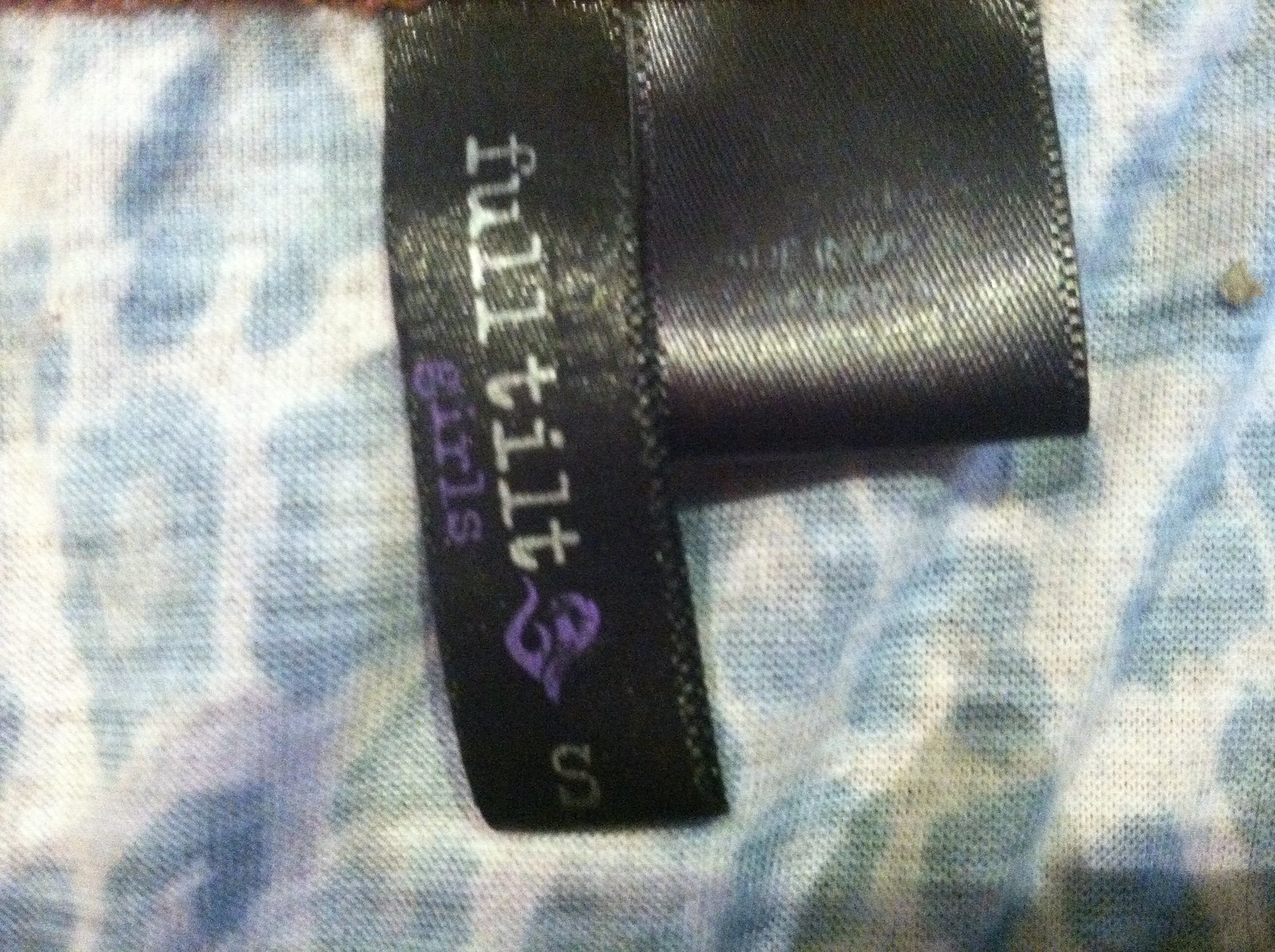In this horizontal, rectangular image, we are presented with a close-up view of the interior of a garment, possibly a sweater or jacket, revealing its tag and fabric lining. The fabric features an animal print design in shades of blue, black, and white, viewed from the inside out. Two black tags are prominently visible at the top center of the image. 

The tag on the left is black and exhibits silver and purple text that reads "Full Tilt Girls," accompanied by a decorative purple scroll design. This tag also indicates the size with a letter "S" for small. 

The second tag, positioned to the right, appears to have been subjected to repeated washings, which has rendered its text significantly faded and illegible. The overall scene highlights the intricacies and wear of the garment's interior details.